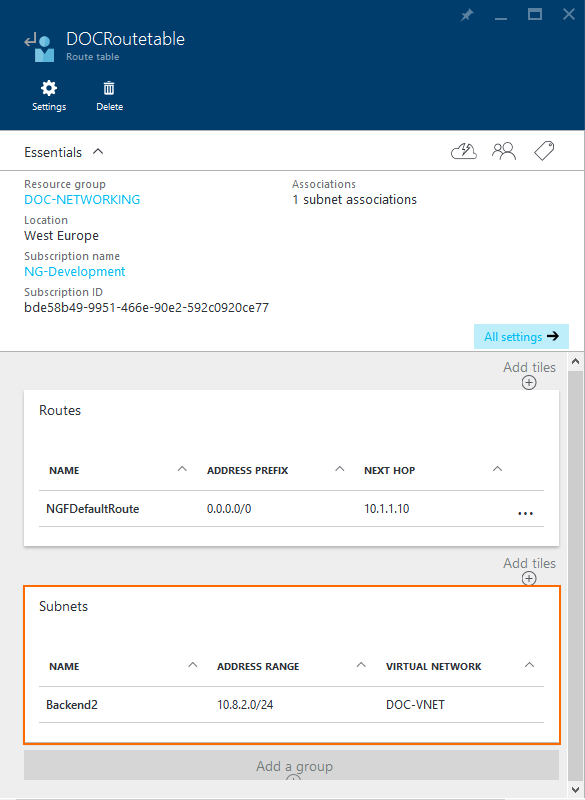This image is a screenshot of a web interface, presented with detailed elements and clear visual hierarchy. On the upper left corner, there is a blue header with the website’s name "DOC Routable Route Table" inscribed. Adjacent to the text is a logo consisting of a blue circle alongside two geometric blue shapes, and a gray arrow pointing left. 

In the upper right corner, an 'X' icon is visible, indicating a close function. Below this, on the left side, are the settings and trash/delete icons. The main content area below these icons features a white background title "Essentials" followed by the subcategories "Resource Group" and "DOC Networking" written in blue text.

To the right of these elements is a section titled "Associations," highlighting "One Subnet Association." Further down, the location is specified as "West Europe," and the "Subscription Name" is given as "NG Development." The "Subscription ID" is displayed in blue text as "BDE58B49-9951-466E-90E2-592C0920CE77." 

At the bottom right corner, there is a blue action box labeled "All Settings," accompanied by an arrow pointing to the right, indicating further navigation or options.